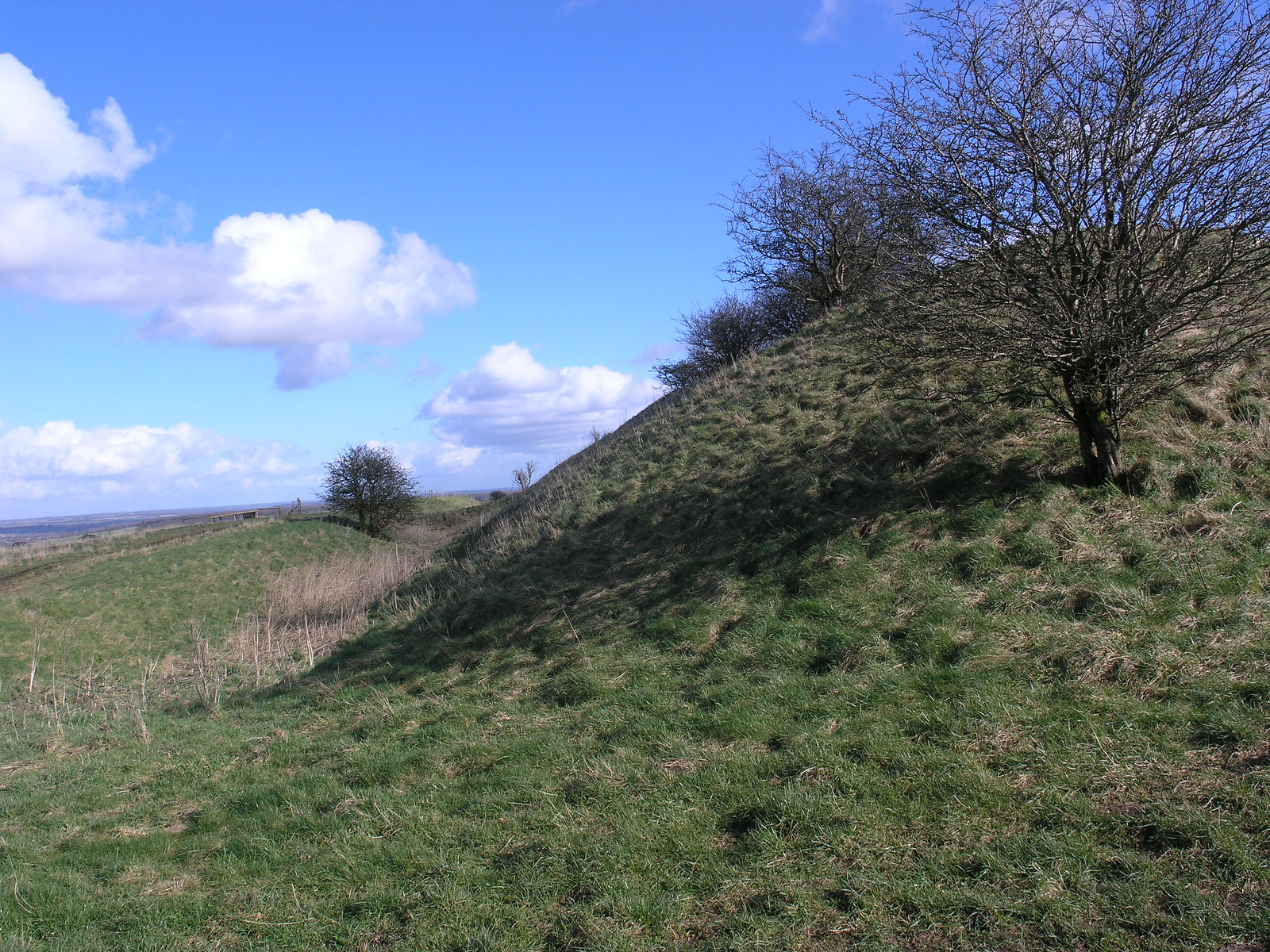The image depicts a tranquil, idyllic countryside scene captured on a bright midday with a light blue sky adorned by marshmallow-like clouds. Central to the picture is a small, gently sloping hill, rising up to about 40 feet, easy to traverse with its light curve. The hill is flanked by tall, unmown grass that sways in the wind, some patches appearing dry. Scattered across the scene are a few barren trees: two atop the hill and one further down the field, all of which seem dry as if their leaves have crusted off. In the background, there are additional, but less prominent, rolling hills. Overall, the green grass is in the process of rejuvenation, with a mix of fresh growth and lingering brown patches. The absence of people or animals adds to the serene and undisturbed nature of the landscape.